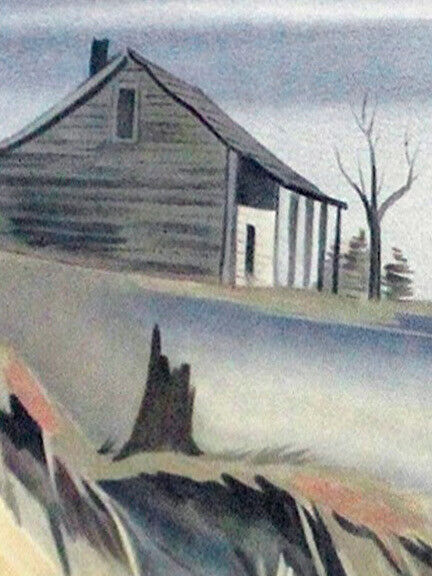This detailed artwork, seemingly created using pastels on paper, depicts a Depression-era homestead or barn, viewed primarily from the left side. The building, characterized by its warbled roof and crumbled chimney, is painted in light gray tones with sections of faded off-white, revealing weather-worn wooden boards beneath. The structure's dilapidated state is evident, with various colorations of black and greens highlighting individual boards. There is a distinctive black door surrounded by a small white wall area at the front, flanked by three light gold pillars and a single dark pillar supporting the roof’s edge. To the right of the house stands a notable barren tree, stripped of all leaves. The ground in the scene is largely barren, featuring abstract rocky elements and minimal grass. A tree trunk, possibly from a long-dead tree, emerges from the ground near the homestead. The background sky transitions from light to dark gray, adding to the somber, nostalgic atmosphere of the image.